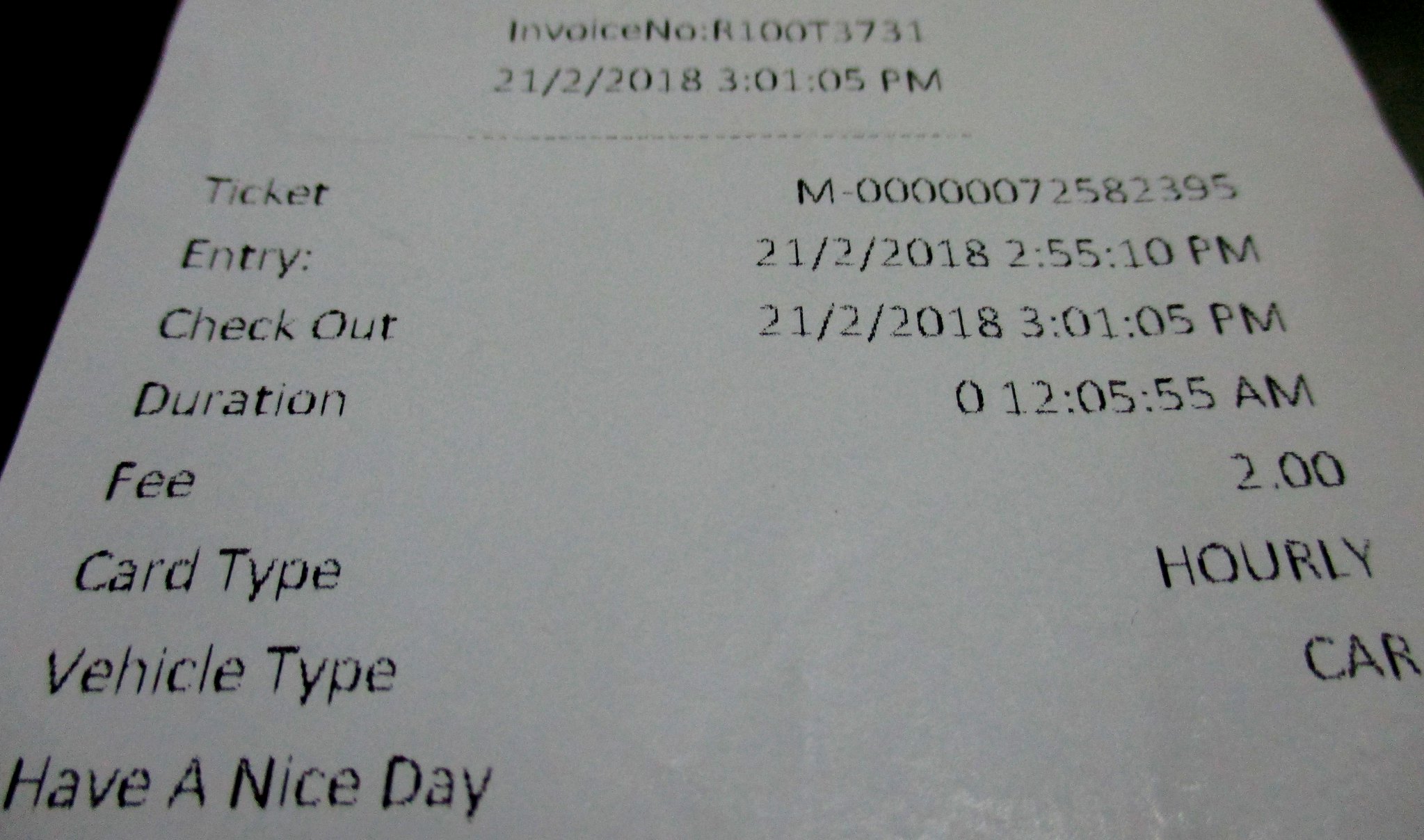This rectangular photograph depicts a simple, zoomed-in invoice set against a white background with black print. The top of the invoice prominently displays "Invoice Number R100T3731," dated "21-2-2018" at "3:01:05 PM." The document is organized into two columns. Down the left-hand side, it lists categories: Ticket, Entry, Checkout, Duration, Fee, Card Type, Vehicle Type, and a courteous "Have a Nice Day" at the end. The right-hand side provides corresponding details: Ticket number "M-00000072582395," Entry date and time "21-2-2018 at 2:55 PM," Checkout date and time "21-2-2018 at 3:01 PM," Duration "01:05:55," Fee "$2.00," Card type "hourly," and Vehicle type "car." Despite the low lighting, all text on the invoice is clearly legible, highlighting its straightforward and functional design.